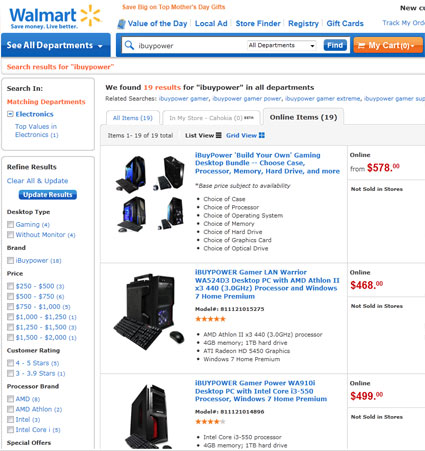A screenshot from Walmart.com showcases search results for the brand "iBuyPower." At the top, the familiar Walmart branding is displayed, featuring the blue background with the characteristic white flower logo and the yellow flower shape to the right. The website layout appears straightforward, with separate sections for navigation and search filters.

On the left-hand side, a vertical box offers options to search within the Electronics Department, highlighting categories like "Top Values in Electronics." Below this, a refinement box allows users to filter by desktop type, brand, price, customer rating, and processor brand.

To the right, the page displays a grid view of 19 search results for iBuyPower products. Visible are three primary results:

1. **iBuyPower Build Your Own Gaming Desktop Bundle**: This option allows customers to customize their gaming desktop by choosing various components including the case, processor, memory, and hard drive. The item is marked with a red "Online" label and priced starting from $578. It is noted as "Not sold in stores."

2. **iBuyPower Gamer LA Warrior Desktop PC**: This listing features a complete setup with a keyboard and desktop, powered by an AMD Athlon II processor and pre-installed with Windows 7 Home Premium. It is priced at $468 and is also "Not sold in stores."

3. **iBuyPower Gamer Power PA910i Desktop PC**: The third result displays just the desktop unit and is priced at $499.

Each product image provides multiple viewing angles, allowing potential buyers to scrutinize the design and features of the computers on offer.